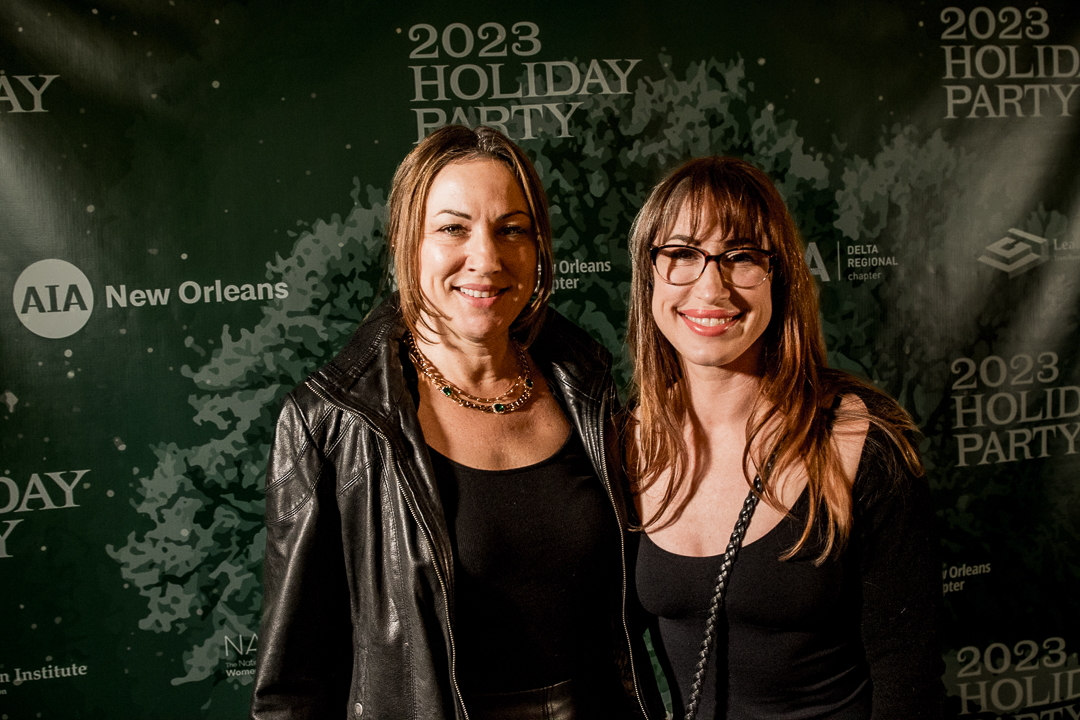In this waist-high photograph taken at the AIA New Orleans 2023 Holiday Party, two fairly young, golden blonde-haired women, appearing to be in their 30s, are posing side by side against a large banner. Both women are dressed in black outfits. The woman on the left, slightly taller, is wearing a black low-cut top paired with a black leather jacket and a double bead necklace. Her hair is styled to neck length. The woman on the right is sporting a low neckline black top without a coat and has something hanging on a long lanyard around her neck. She is accessorized with large-rimmed glasses and her hair falls below her shoulders. They have their arms around each other's backs and are smiling. The decorative banner behind them features repeated white text stating "2023 Holiday Party" interspersed with various corporate logos, some including the words "AIA" and "New Orleans," against a background that appears to depict snow-covered trees or leaves.